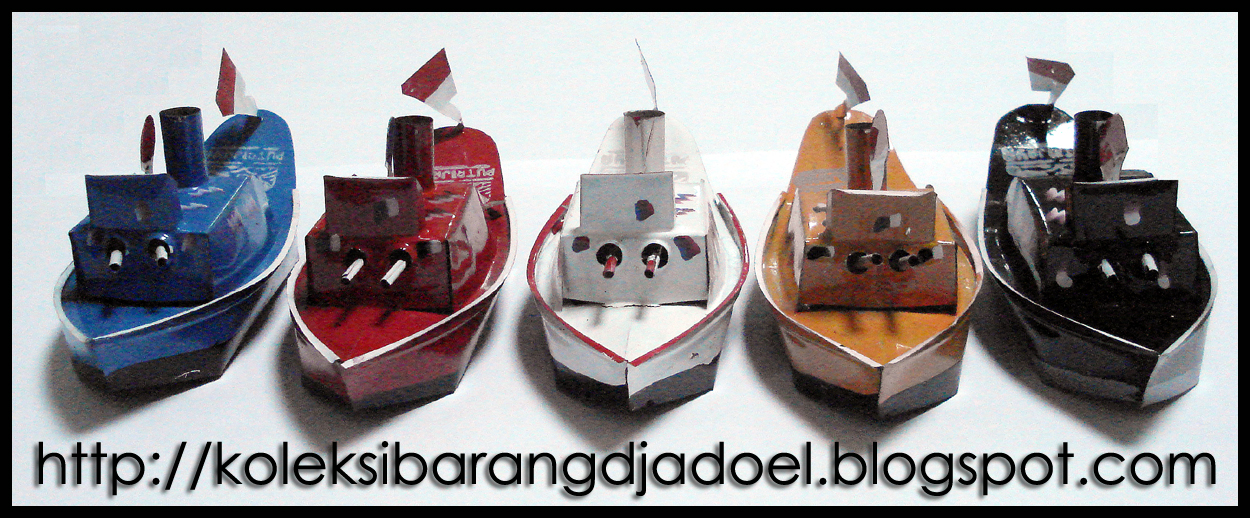This is a professional landscape-format photograph featuring five model tugboats arranged in a row on a white surface. The boats are painted in blue, red, white, orange (or brown), and black, with each one featuring black paint on the part that would be underwater. All the tugboats are designed with two cannon-like guns at the front and a chimney stack on top of the deck. They also display flags at the back, each with two horizontal stripes—red on top and white on the bottom. Across the bottom of the image, there is a blog address in a language that seems to be Dutch or Norwegian, reading "http://koleksibarangajadoel.blogspot.com." Despite the different colors, the tugboats share an identical design.